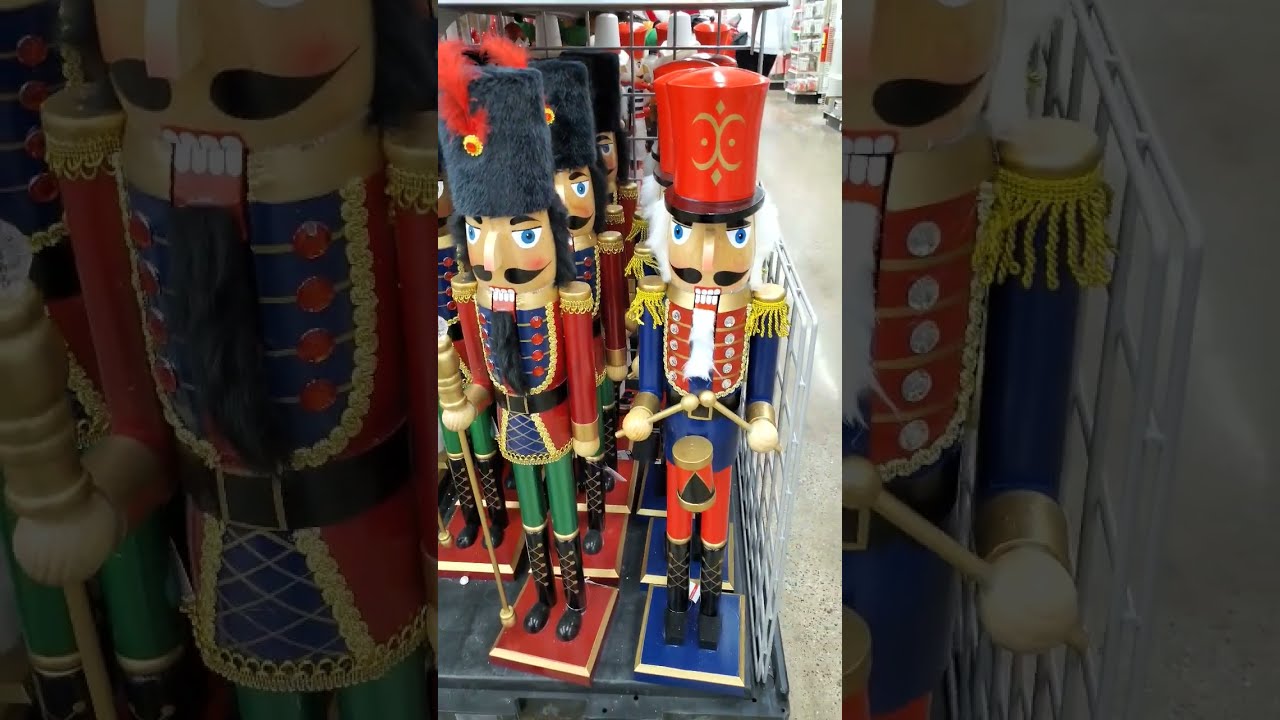The image features a vibrant display of large nutcrackers standing in rows, part of a festive shopping center presumably decorated for Christmas. These nutcrackers are adorned in colorful and intricate outfits. One on the far right wears a red hat, red pants, black boots, and has yellow tassels on the shoulders of his red jacket decorated with gold buttons. He holds a little drum and drumsticks. Another notable nutcracker, positioned centrally, boasts a blue jacket, red pants, and a red hat with white hair peeking out. He has a gold belt buckle and drumsticks crossed in his hands. On his platform is blue. Nearby, a nutcracker with a furry black hat adorned with a red feather stands guard. This one is dressed in a red jacket with yellow shoulder pads, green pants, and dark brown boots. The very center of his chest is blue with red buttons, and he stands on a red platform, holding a gold staff. The setting clearly indicates they are in a bustling store aisle, as evidenced by visible shelves and merchandise in the background. The nutcrackers appear to be mounted on a pallet with a guardrail in front, against the backdrop of a shiny marble floor and bright lighting, capturing the essence of holiday shopping.